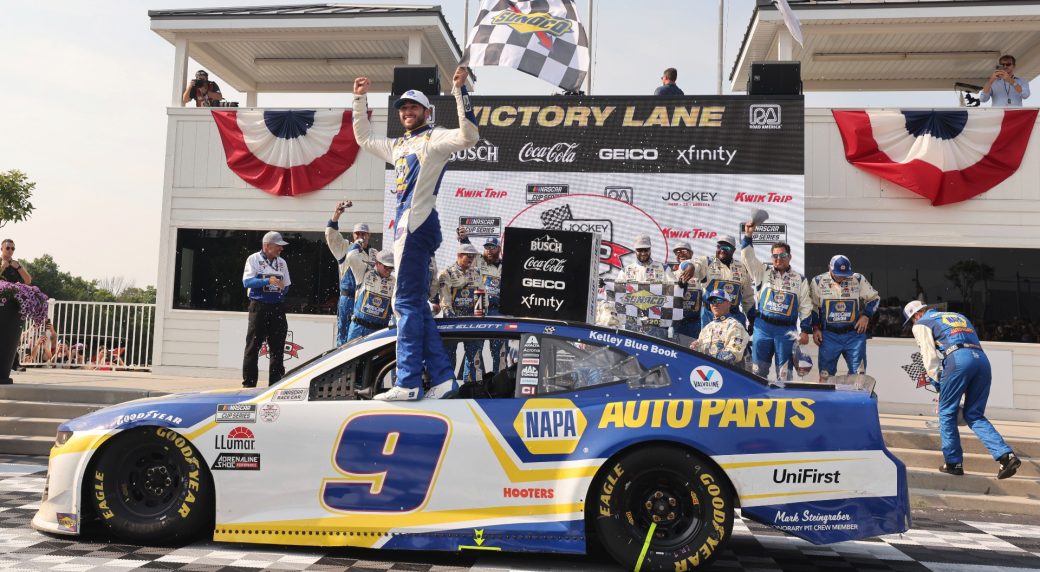The image captures a jubilant moment at a NASCAR race. At the center is a vibrant blue, yellow, and white race car bearing the number 9 and adorned with various sponsors such as Napa, Hooters, UniFirst, Goodyear, Kelly Blue Book, and Sunoco. The driver, dressed in a blue jumpsuit and white long-sleeve shirt with a white cap, stands triumphantly on the edge of the car's window, both arms raised at 90-degree angles and a broad smile on his face. He holds a Sunoco checkered flag, symbolizing his victory. Behind him, the scene is further embellished by a white building featuring red, white, and blue bunting on two terraces. The central balcony displays the words "Victory Lane" painted on the block wall. The background is populated by a group of men in mechanics' jumpsuits matching the blue of the car, posing proudly. Additionally, there are various advertisements from Bush, Coca-Cola, Geico, and Xfinity visible around the Victory Lane area. Photographers occupy the stands, capturing this victorious moment.